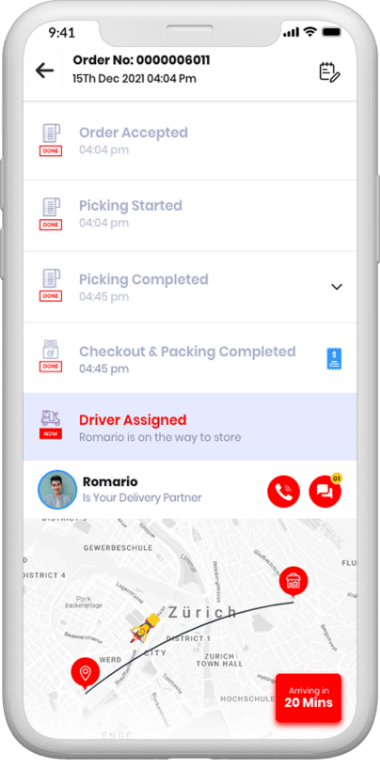The image showcases a smartphone displaying a delivery tracking interface against a white background. The screen shows a delivery update with several details:

- **Top Section**: The background of the app page is white. At the top, black text reads, "Alter number: 0000006011, 15th December 2021, 04:04 PM." There's an 'Edit' button on the top right and a 'Back' button on the top left.
- **Status Updates**: Below the alter number, light navy text states, "Alter accepted, 04:04 PM." Another entry, written in Danish red, includes a small icon of a paper.
- **Process Timeline**:
  1. **Step 2**: "Picking started at 04:04 PM."
  2. **Step 3**: "Picking completed at 04:45 PM."
- **Driver Assignment**: The text at the bottom of this section states, "Driver assigned." This text is also in red. It further mentions, "Romario is on the way to store," indicating the driver’s name.
- **Driver and Delivery Information**:
  - A map of Zurich is displayed at the bottom, showing Romario’s route.
  - A profile section features Romario's information, including his role as a delivery partner.
  - Additional details say Romario is arriving in 20 minutes.
  - There are red call and chat buttons on the right side for contacting the driver.
- **Driver’s Vehicle**: The map displays an icon of Romario on a yellow bike. He is wearing yellow.

Overall, the detailed interface keeps the user updated on the delivery status, driver’s journey, and provides options to contact the driver if needed. The real-time map ensures transparency in tracking the delivery’s progress.